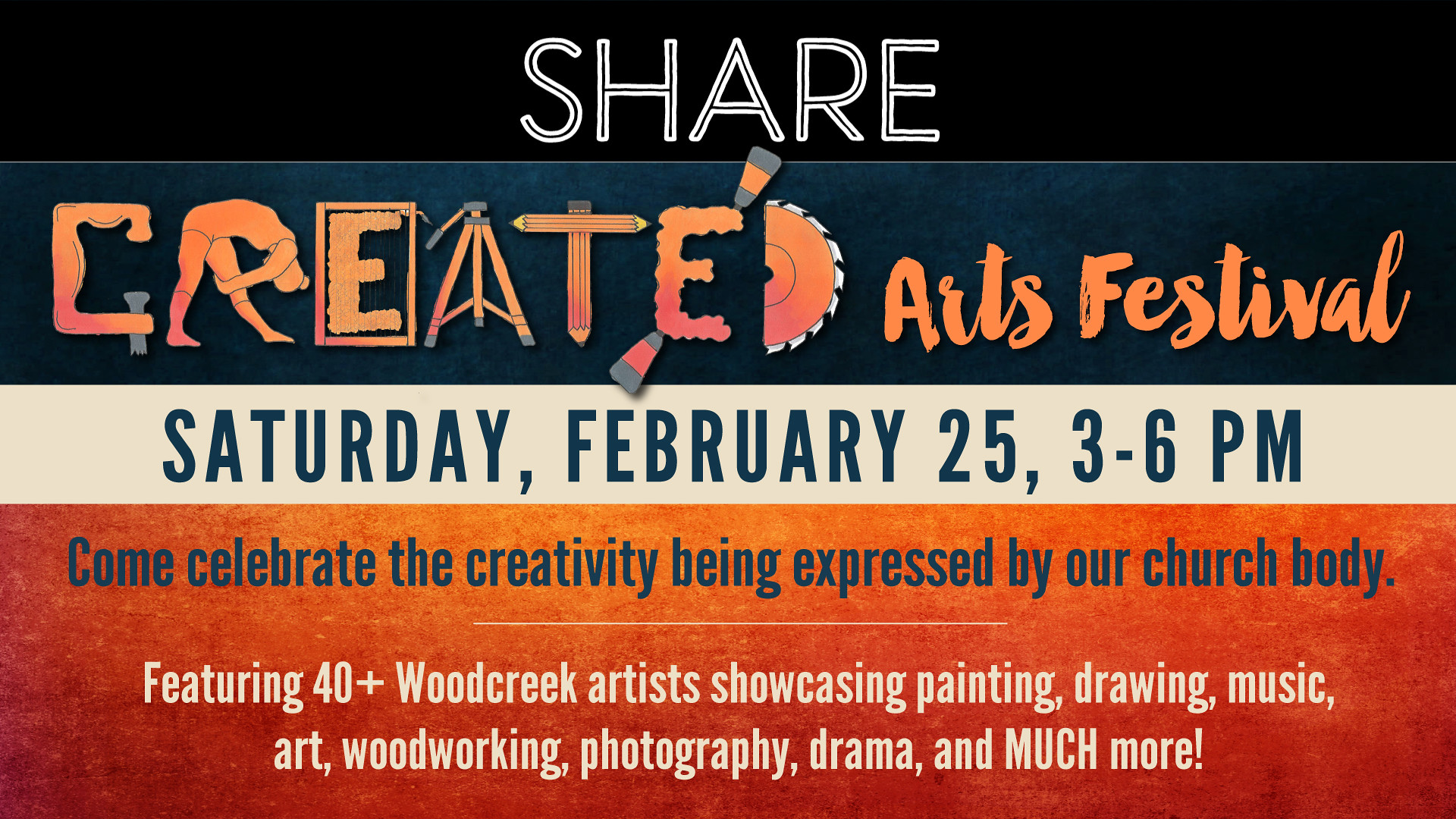This vibrant and eye-catching advertisement for the "Created Arts Festival" invites everyone to celebrate creativity on Saturday, February 25th, from 3 to 6 PM. The poster is divided into visually distinct sections, each with its own color scheme to emphasize various details. 

At the top, the word "SHARE" stands out in uppercase black letters with white outlines, against a black background. Directly below, a blue section boldly announces "CREATED ARTS FESTIVAL," with each letter uniquely crafted from various elements and objects: a flexing arm forms the "C", a person bending over shapes the "R", the first "E" is framed by a square, the "A" is crafted from a tripod or camera, the "T" from a pair of pencils, the second "E" with jagged edges, and the "D" from half a saw blade. The words "ARTS FESTIVAL" follow in a creative, cursive script with green or orange letters.

A lighter white section beneath displays the event details in blue letters: "SATURDAY, FEBRUARY 25th, 3 to 6 PM." The bottom section, blending orange and yellow hues, conveys the celebratory message in grey letters: "COME CELEBRATE THE CREATIVITY BEING EXPRESSED BY OUR CHURCH BODY." Below a white line, grey text also highlights the event’s offerings: "FEATURING 40 PLUS WOODCREEK ARTISTS SHOWCASING PAINTING, DRAWING, MUSIC, ART, WOODWORKING, PHOTOGRAPHY, DRAMA, AND MUCH MORE!"

The overall design is described as colorful and creative, featuring segments with black, blue, and orange backgrounds, and alternating between white, blue, and grey text to draw attention and provide information clearly and artistically.